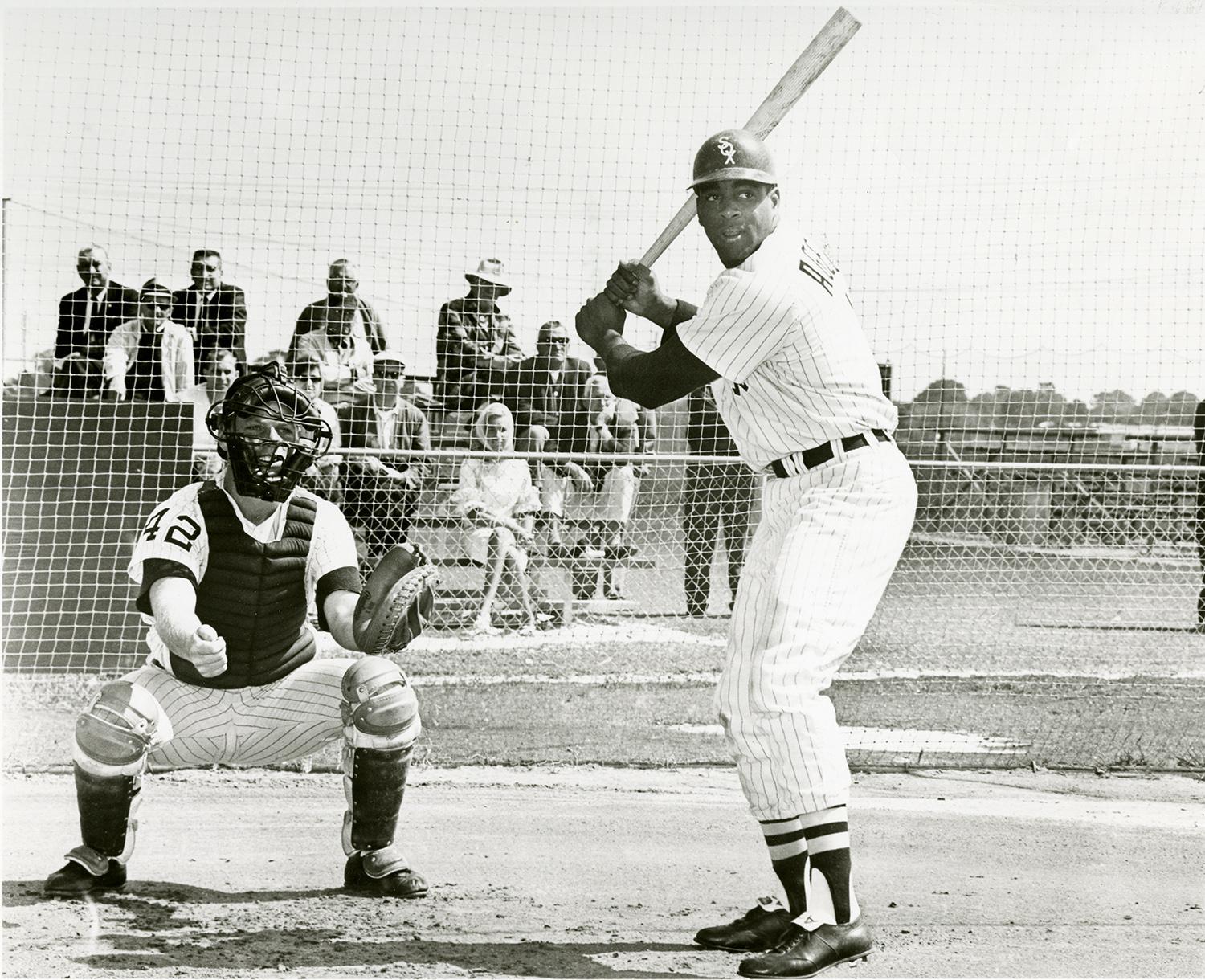In this black and white photograph, we see an intense baseball moment captured as an African American batter stands at home plate, poised to swing. He is outfitted in a white uniform with dark stripes and black leather cleated shoes, wearing a black hard plastic helmet emblazoned with the white letters "SOX." His arms are raised chest high, gripping the bat behind him as he focuses intently on the unseen pitcher ahead. The name on the back of his uniform starts with the letter "A," though it is difficult to discern clearly.

Directly behind the batter, the catcher is squatted down, fully geared in protective equipment including a face mask and a black vest with the number 42 on the right shoulder. His left hand is covered by a large catcher's mitt, ready to receive the pitch. 

Beyond this dynamic duo, a stringed fence provides a barrier for the group of spectators seated on the bleachers. There are approximately 10 to 15 people watching the game, some wearing sunglasses and hats, with one woman in a light-colored outfit adorned with a light scarf standing out. One individual is observed standing to the right side of the bleachers. In the distance, the scenery includes additional fencing and a backdrop of trees on the right side, with what appears to be a train passing by. The scene effectively captures a lively and detailed moment in this historical baseball game.